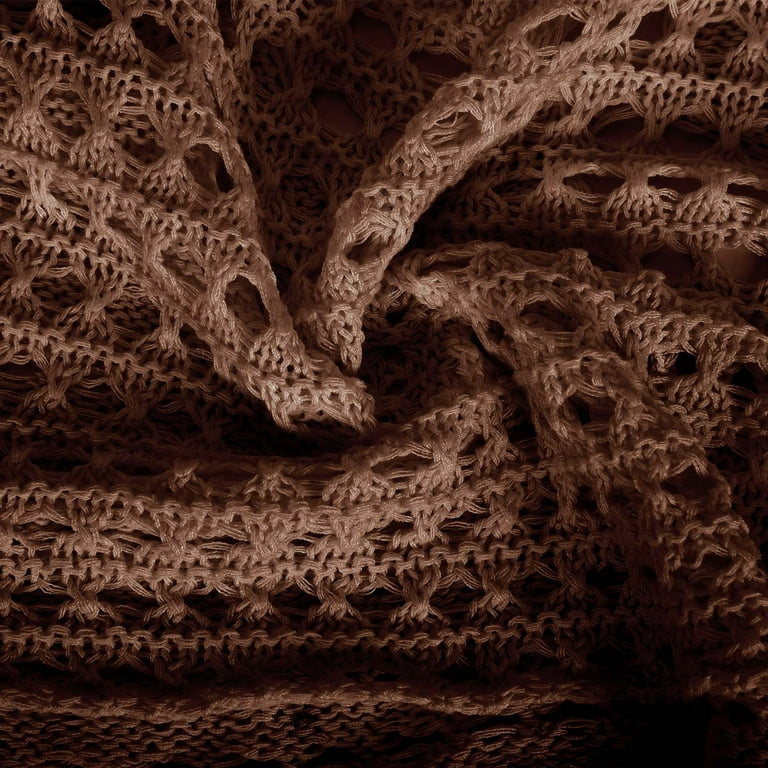The image showcases a detailed close-up of a woven fabric, possibly wool or a loosely knitted material resembling a sweater or a blanket. The fabric, light brown in overall color, displays a gradient effect where it appears lighter on the top and transitions to a darker brown towards the bottom. The texture is characterized by numerous small, circular holes, creating a mesh-like pattern that highlights the intricate threading. This knitting or weaving is well-constructed, with a twisted appearance in the central area where more light is focused. Shadows accentuate the piece, especially in the lower right corner where the fabric scrunches together, enhancing the brown tint of the shadowed areas. There’s a slight fold at the top of the material, contributing to an organic, slightly rumpled appearance, and the entire image, while detailed, doesn't feature any background elements, keeping the focus entirely on the textured fabric.